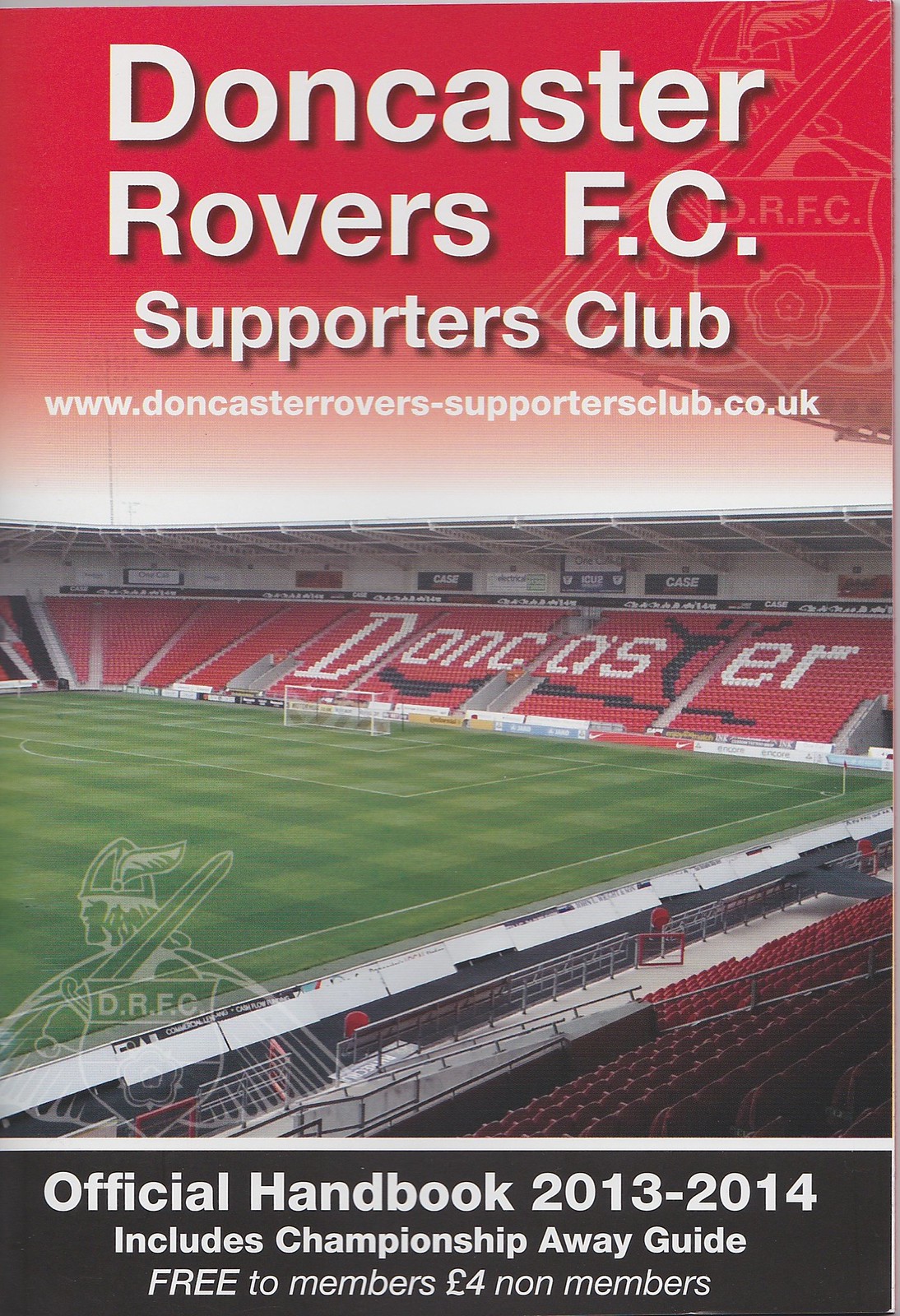The cover of the Doncaster Rovers FC Supporters Club official handbook for the 2013-2014 season is detailed and visually structured in a vertical rectangular layout. At the top, against a red background with white lettering, it proudly states "Doncaster Rovers FC Supporters Club," followed by their web address. The centerpiece of the cover features a panoramic photograph of the Doncaster stadium, showcasing an empty green soccer field with stands that spell out "Doncaster" in various colored seats. Adding to the design, a subtle Viking logo is faded into the lower left corner of the photograph. Below this central image, a black horizontal stripe features prominently, again in white letters, the text "Official Handbook 2013-2014," along with additional details: "Includes championship away guide, free to members, £4 for non-members." This structured layout encapsulates both the pride in the club and essential information for the season ahead.